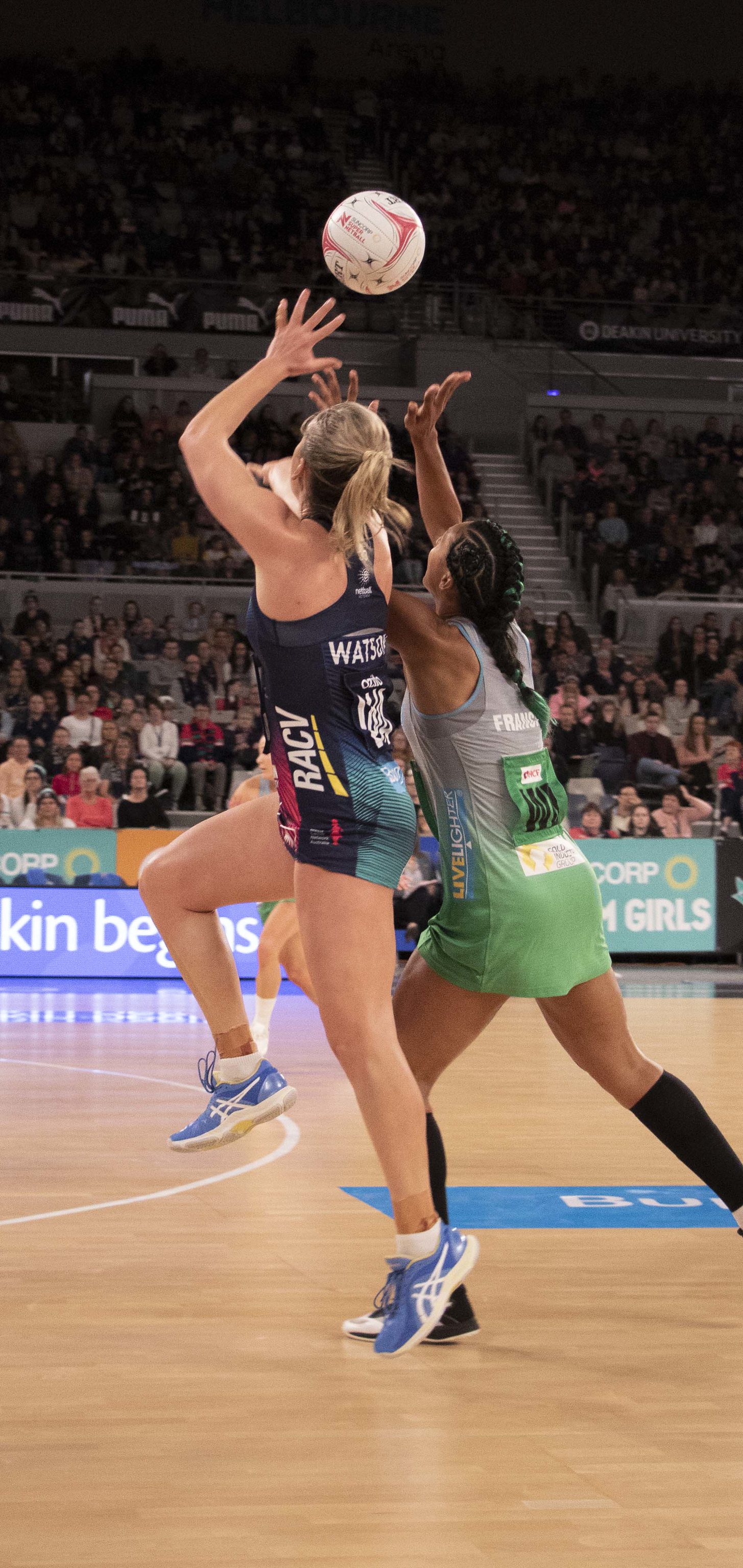This tall, rectangular photograph captures an intense moment from a women's volleyball game within a spacious arena. The arena features several densely packed rows and levels of bleachers, with spectators closely watching the action. The light brown hardwood floor of the court, marked with blue and white paint, stretches out across the lower half of the image. Various banners and advertisements, in colors like green and purple, are visible at the edge of the court.

In the foreground, two women are leaping into the air, both with their arms outstretched, attempting to hit a white volleyball accented with red stripes. The woman on the left is a Caucasian athlete wearing a navy blue tank top and shorts adorned with various advertisers' names, including a notable "RACV" logo. Her right leg is bent upwards, while her left leg is almost touching the ground. The woman on the right has black skin, long black braided hair with green-dyed sections, and is dressed in a green and gray uniform. She also wears black knee socks and sneakers. Both athletes are fully focused on the ball, displaying their athletic prowess in the heat of the match.